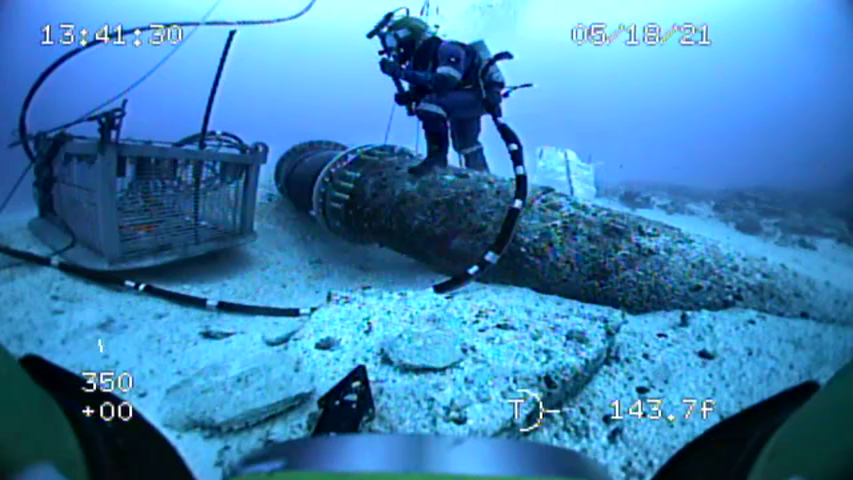The black-and-white underwater photograph, seemingly taken with a grainy camera, showcases a detailed scene at the ocean floor. A lone scuba diver, equipped with a scuba mask, oxygen tank, and black hose extending off-camera, is seen navigating the terrain. The diver appears to be investigating or climbing over ruins that could be part of a decayed shipwreck or an old, corroded structure, possibly fallen from a ship or plane. Among the wreckage, there are discernible elements like encrusted metal links, a corroded pipe, and a large metal container whose purpose remains unclear—potentially a trap or a collection container. Nearby, a white cage-like structure with black ropes and additional debris such as pieces of a large metallic object lie scattered. The seabed features whitish sand interspersed with rocks or coral, under a top layer with a bluish hue. Notable time and date stamps are visible: "51821" at "1341 30" on the upper right and different numbers like "350 + 0 0" on the lower left and "143.7 F" on the bottom right.